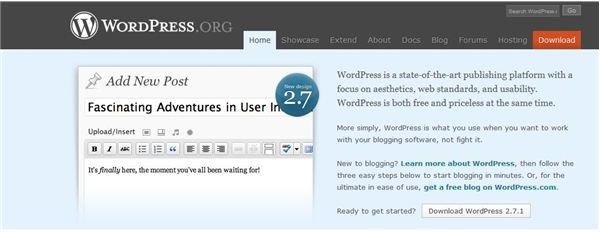### Detailed Descriptive Caption:

This image is a screenshot of the homepage from WordPress.org. At the top of the page, the WordPress logo is prominently displayed: "WordPress" is written in white letters accompanied by a symbol that features a 'W' in black, encapsulated by a white circle with a surrounding white ring. Right next to the logo, "WordPress.org" is shown in a gray font.

The navigation menu beneath the logo includes several options: Showcase, Extend, About, Docs, Blog, Forums, and Hosting. There is also a conspicuous red box labeled "Download." Above this download button, the search bar is labeled "Search WordPress."

The page background is a visually calming blue. Part of the homepage features a sticky note element pinned at the top with a push pin, reading "Add New Post". The title "Fascinating Adventures in User IN" is written on this note, accompanied by a teal circle that has "2.7" in white letters and numbers.

Below the title, the options "Upload/Insert" are provided with four icons: a musical note symbol, a square with a smaller square inset, a square with a smaller square situated in the upper left corner, and a circular icon. The text editor interface displayed has a gray background and features a comprehensive set of text formatting buttons, including options for bold, italics, bullet points, quotes, and text alignment (left, center, right).

Within the main content area, there is a message that reads, "It's finally here, the moment you've all been waiting for!" To the right of this message, a descriptive text about WordPress states: "WordPress is a state-of-the-art publishing platform with a focus on aesthetics, web standards, and usability. WordPress is both free and priceless at the same time. More simply, WordPress is what you use when you want to work with your blogging software, and not fight it. If you're new to blogging, learn more about WordPress." The phrase "learn more about WordPress" is highlighted in green.

Furthermore, the page encourages users with the text: "Follow the three easy steps below to start blogging in minutes or, for the ultimate in ease of use," followed by the green text, "Get a free blog on WordPress.com." Finally, at the bottom of this section, there is the prompt "Ready to get started?" followed by a white rectangular button that says, "Download WordPress 2.7.1."